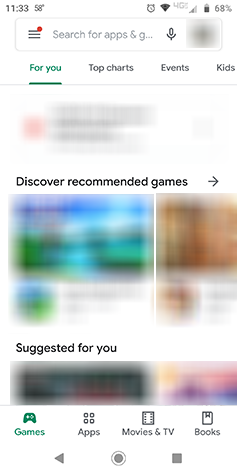In the top left corner, the image displays the number "1133," presumably indicating the time, and a temperature reading of "58 degrees." On the top right, there is an alarm clock icon, a signal strength indicator, a "4G" label, and a battery icon showing a 68% charge. Beneath these icons, there is a search field labeled "Search for apps and G," with a microphone icon for voice search. The right end of this search field is obscured by a blurry, gray image, making it difficult to decipher the remaining content.

Below the search field are headings labeled "4U," "Top Charts," "Events," and "Kids." The "4U" is highlighted in green, indicating it is currently selected. Under this heading, there is a blurry image featuring something red—possibly an icon—accompanied by some text.

Further down, a large, bold heading reads "Discover Recommended Games," with an arrow pointing to the right. Various blurred, colorful images appear beneath this heading. Following that, there is another section titled "Suggested For You," containing one or two images that are also blurred and unclear.

At the very bottom, a row of four icons with labels reads "Games," "Apps," "Movies & TV," and "Books," with the "Games" icon currently selected.